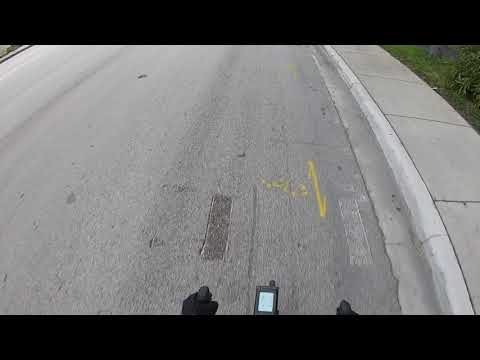This photograph, taken from the perspective of a bicyclist, features an almost animated feel with black bars on the top and bottom framing the main image. At the very bottom, you can see the bicyclist's handlebars, gripped by hands in black gloves, and a small, barely visible digital screen likely for tracking speed and mileage. The roadway extends horizontally across the frame, marked by varying textures and shades of asphalt. A prominent yellow line with shorter lines protruding from its top and bottom runs vertically in the center. On the right side of the road, there is a concrete curb with a sidewalk segmented into squares, followed by a stretch of green grass and possibly some tree foliage in the top right corner. The upper left corner also hints at a curb on the opposite side. The image is devoid of other vehicles, animals, or people, with predominant colors being tan, yellow, and white.